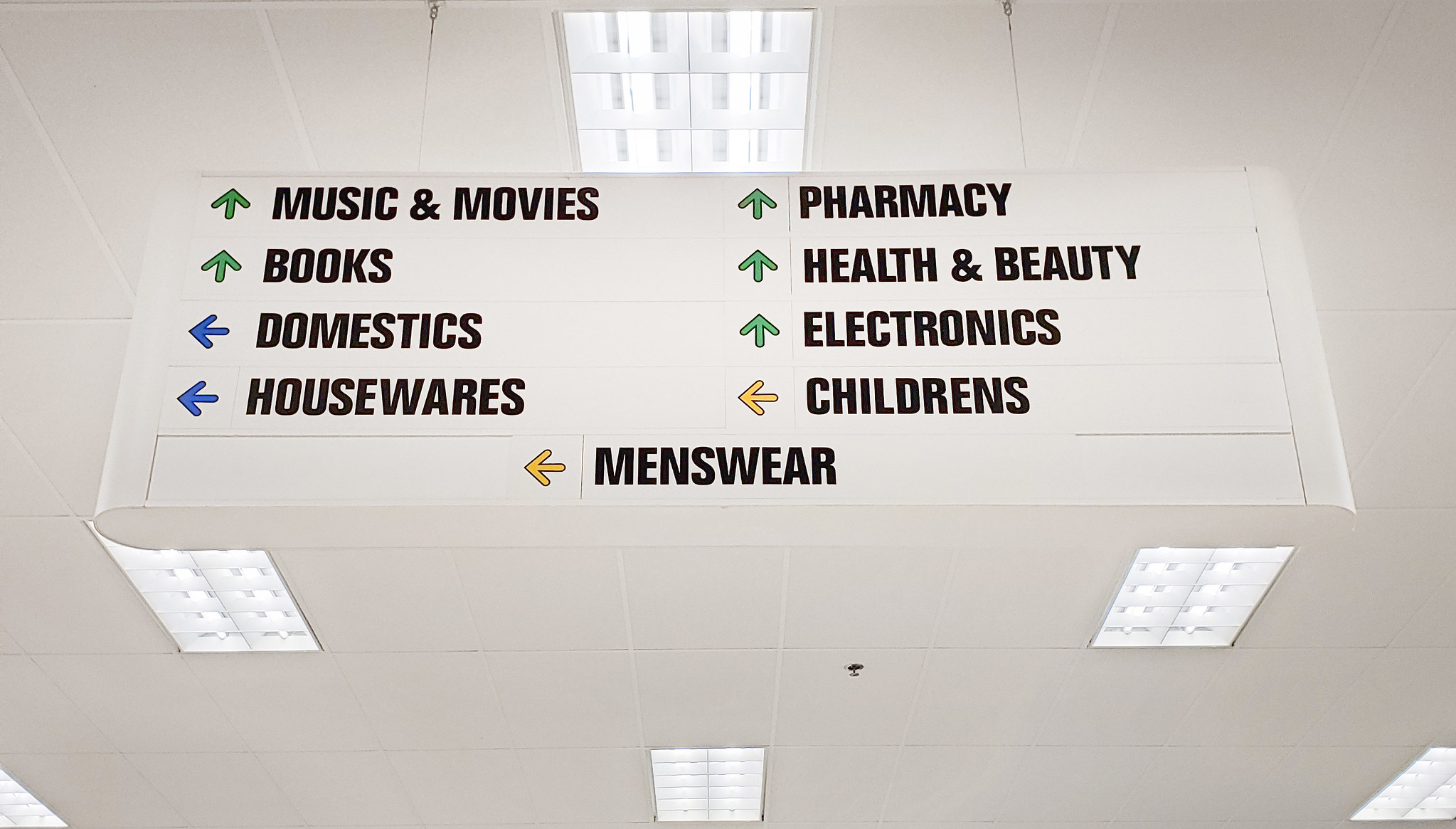The image captures the interior of a store, showing a white ceiling adorned with a grid of square tiles and several rectangular light fixtures. Suspended from the ceiling by two wires is an elongated, rectangular sign with rounded edges that serves as a directory for various departments within the store. The sign is white with distinct, color-coded arrows and text indicating the locations of different aisles. 

Green arrows pointing up direct customers to "Music and Movies," "Books," "Pharmacy," "Health and Beauty," and "Electronics." Blue arrows pointing left guide shoppers to "Domestics" and "Housewares." An orange or yellow arrow on the left points to the "Children's" section, while another yellow arrow at the center bottom directs attention to "Menswear." This sign is a key navigational tool to help customers efficiently find their desired items in the store.